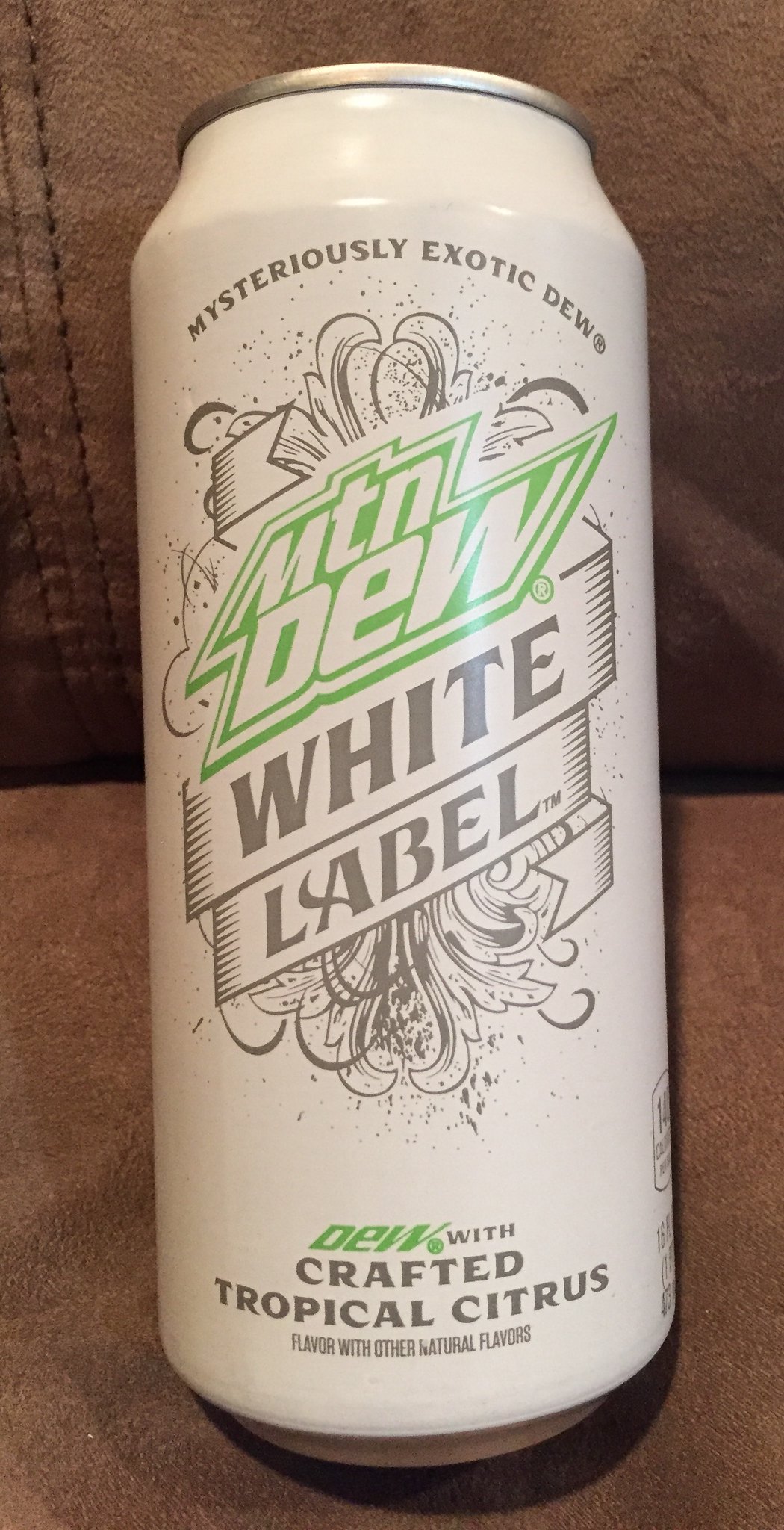This image is a detailed close-up of a 16-ounce can of Mountain Dew White Label, resting on what appears to be a brownish-gray suede or leather surface, showcasing visible stitching in the background. The can primarily features a sleek and ornate white design with the Mountain Dew logo prominently displayed in a bright green color near the center. Above the logo, in an arched, silver text, it reads "Mysteriously Exotic Dew™." Below, in a decorative banner, the text "White Label" is inscribed. Further down, additional descriptions in black or dark gray lettering state, "Dew with Crafted Tropical Citrus Flavor" and "with Other Natural Flavors" in smaller print. The can also includes visible nutritional information on its right side, indicating around 140 calories. Ornate design elements behind the text suggest a lively and festive theme, adding to the visual appeal of this special edition soda can.